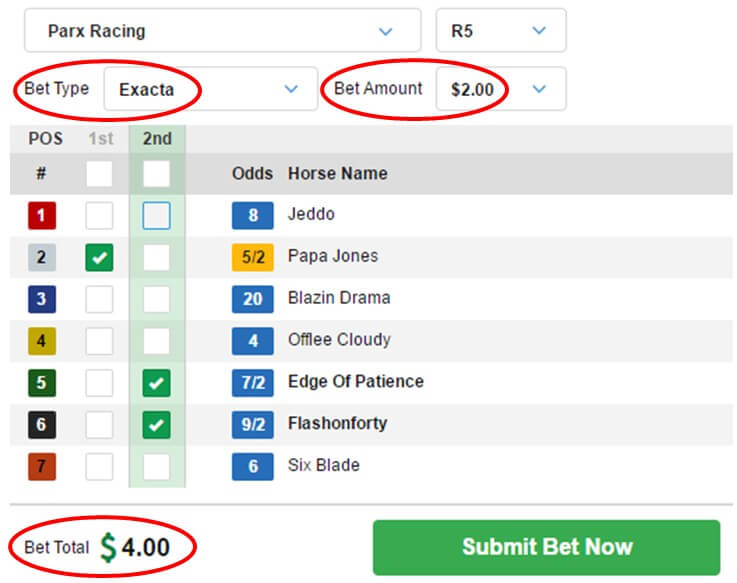This screenshot depicts a webpage from a horse racing website named "Parks Racing." In the top left corner, there's a drop-down menu with various options for navigation. The central part of the page displays detailed information about an ongoing or upcoming horse race. The information includes the current positions of the horses, listed from first to seventh place. Next to each position, the names of the horses and their respective odds are clearly shown. For instance, the horse named "Jetto" has odds of 8, while "Papa Jones" has odds of 5-2, and "Awfully Cloudy" has odds of 4. The webpage is a rich source of information for enthusiasts and bettors who are tracking the race.